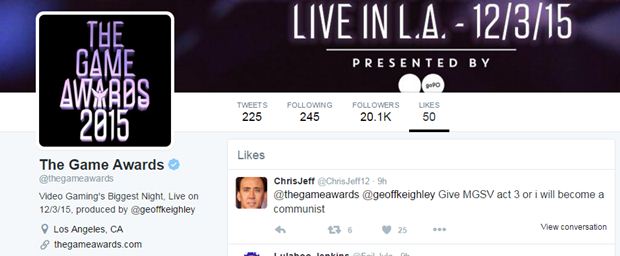The image appears to be a screenshot of a Twitter profile, specifically for "The Game Awards" event held in 2015. At the top of the image, there is a horizontal bar with a gradient that transitions from black to blue to purple, with white text on the right side that reads, "Live in LA, 12-3-15, presented by." In the upper left corner of the image, a black square with a white border contains the text "The Game Awards 2015." Directly beneath this, it's written, "The Game Awards," followed by a blue verification checkmark and the handle "@TheGameAwards." Additional text below reads, "Video Gaming's Biggest Night, Live on 12-3-15, produced by Jeff Kiley, Los Angeles, California."

To the right of this main section, inside a white area, various Twitter metrics are listed: "Tweets 225, Following 245, Followers 20.1K, 50 Likes." Below the "Likes" section, there is a profile picture that appears to be Nicolas Cage. The adjacent text reads, "Chris Jeff, @TheGameAwards," followed by the tweet, "Jeff Kiley, give MGSV Act 3 or I will become a communist." Although the image resembles Nicolas Cage, the profile name suggests it might be someone else.